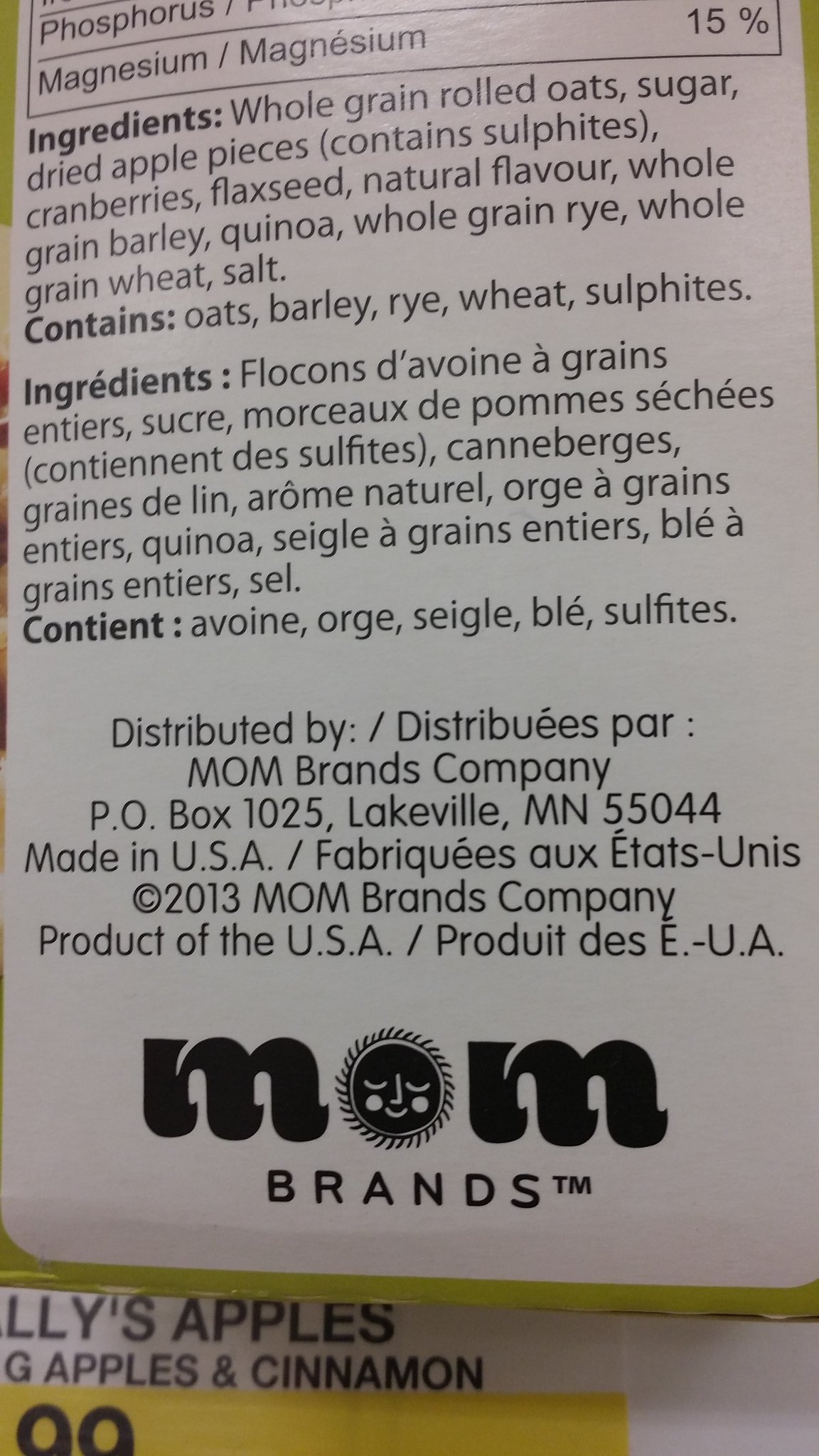This image features the back of a packaged food product, showcasing detailed ingredient information and nutrition facts. At the bottom of the packaging, the nutrition label indicates percentages for minerals such as phosphorus and magnesium, both listed at 15%. The ingredients list includes whole grain rolled oats, sugar, dried apple pieces (with sulfites), cranberries, flaxseed, natural flavor, whole grain barley, quinoa, whole grain rye, whole grain wheat, and salt. The packaging notes allergens, specifying that it contains oats, barley, rye, wheat, and sulfites. The same information is provided in what appears to be French.

Further down, the packaging states that the product is distributed by MOM Brands Company, including an address and the notation "Made in USA 2013". The MOM Brands logo is displayed, featuring a whimsical design where the 'O' is depicted as a sun with closed eyes.

Additionally, there is a close-up image of a shelf label indicating the product variety, "Apples and Cinnamon." Part of the price tag is visible in a yellow section below the label, but it is partially cut off, making the price unreadable.